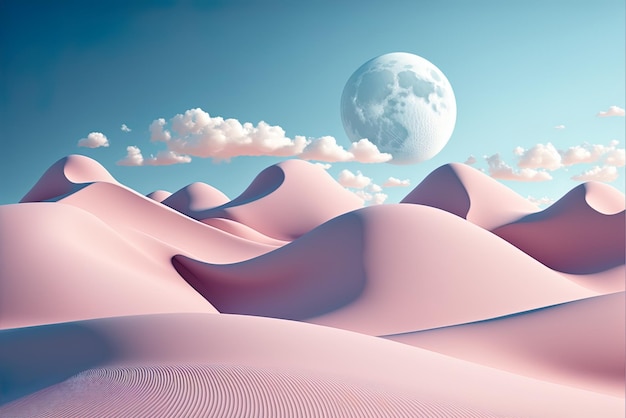The image presents a digitally generated, surreal landscape depicting pink sand dunes that stretch across a desert-like environment without any vegetation or buildings. The sand dunes are unusually smooth, reminiscent of the meticulously raked sand in a Japanese zen garden. Above the horizon, small, fluffy clouds linger in a clear sky, tinted with a subtle pink hue along their undersides. The sky transitions from a light blue in the middle to a darker blue toward the upper left corner. Near the center-right of the sky, a large moon or planet is visible, adding an otherworldly quality to the scene.